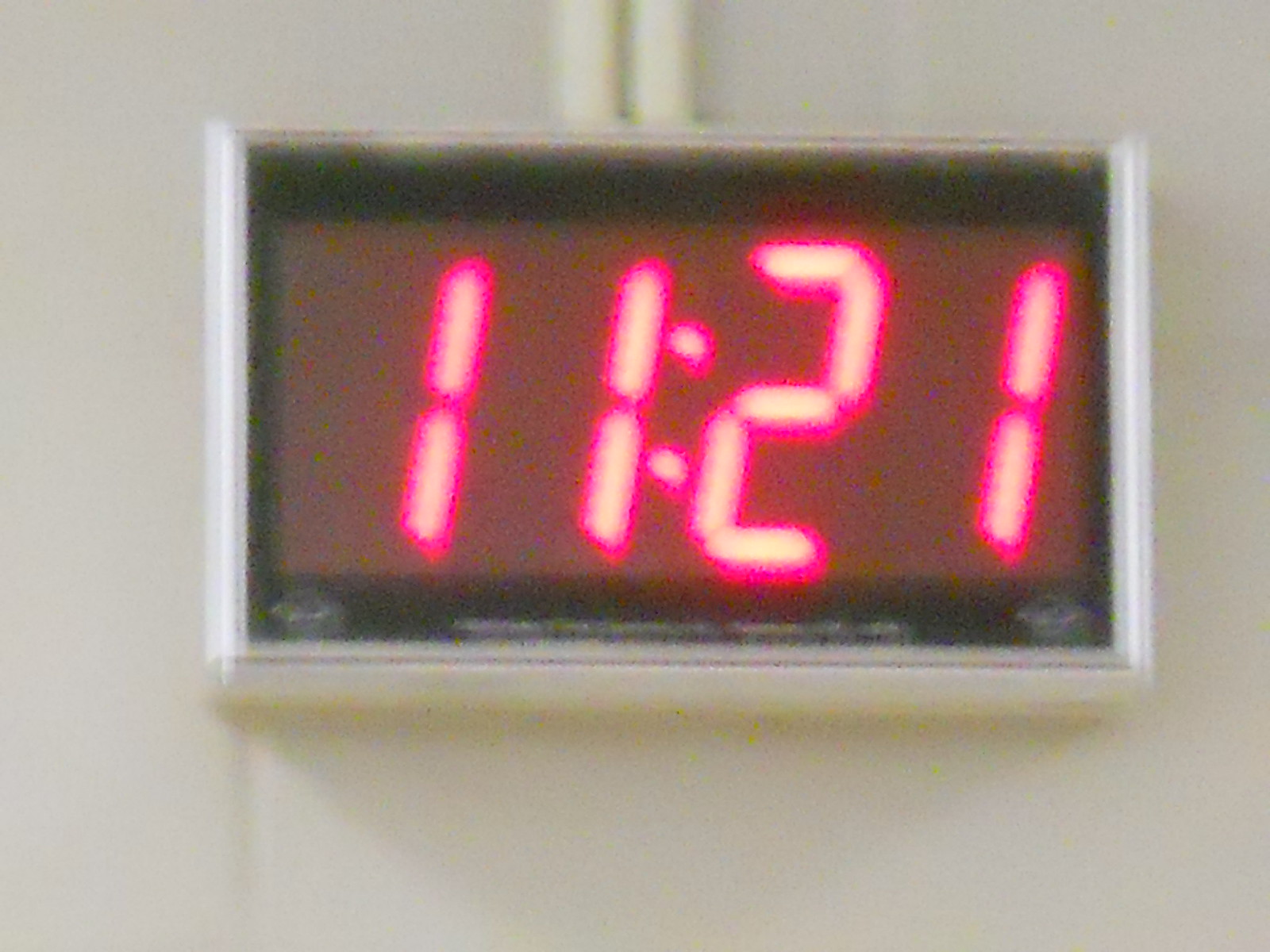This is a slightly blurry close-up image of a rectangular digital clock mounted on an off-white wall. The clock itself has a white frame, within which is a black border. Inside the black border, the clock displays the time "11:21" on a large LCD screen with a maroon background. The digits are created with white lines outlined in pinkish-red, giving a vivid display. Underneath the digits, there is small, unreadable white text on the black trim part. The clock is supported by two cylindrical white poles or pipes that connect to its backside. Additionally, some vague logos can be seen at the bottom corners of the clock. The overall setup juxtaposes a blend of white, black, and maroon hues, making the digital display stand out prominently against the white wall background.